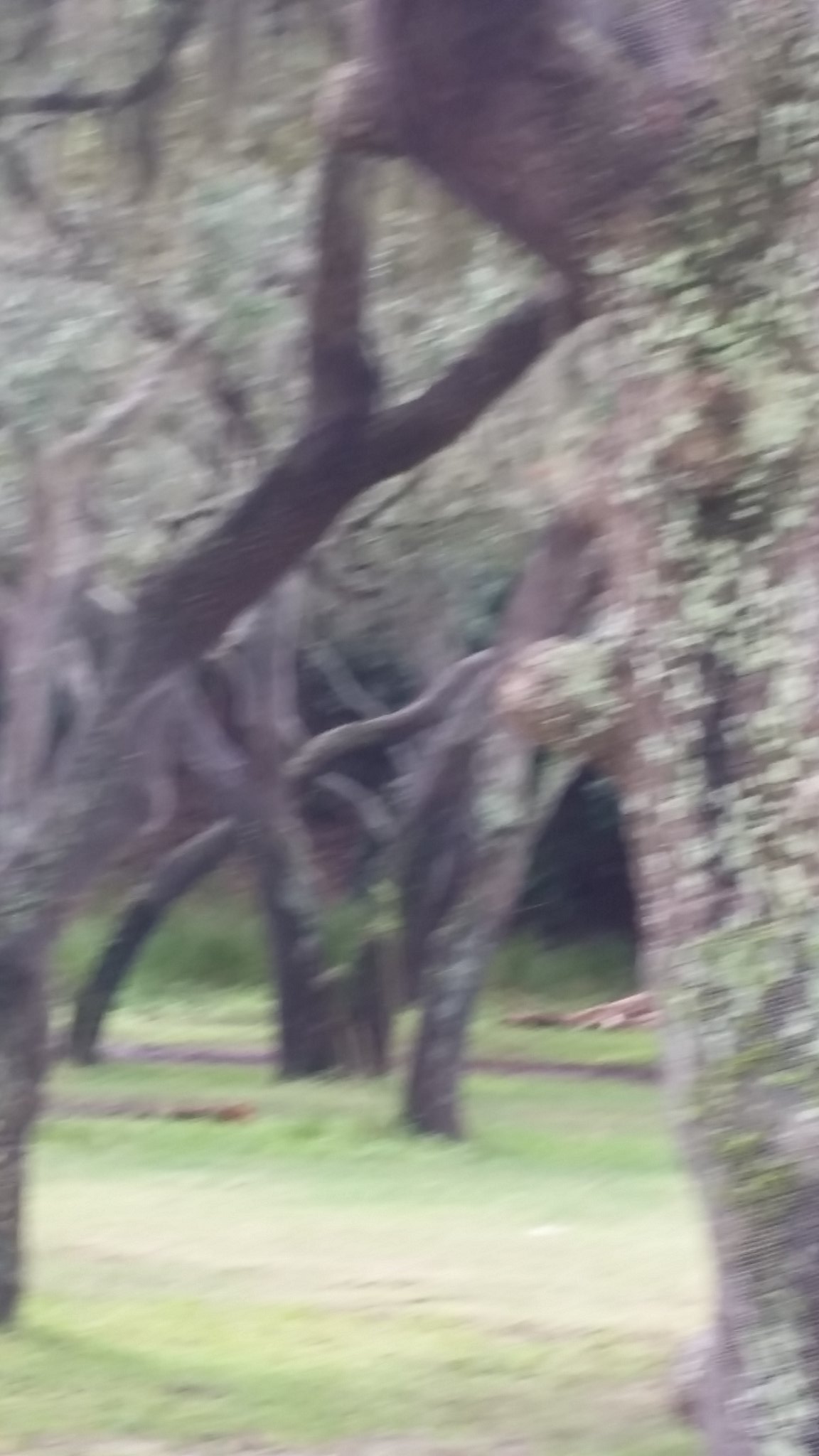The image is a color photograph taken outdoors in a heavily wooded area, though it appears very blurry and some of the colors seem somewhat washed out. We can discern numerous brownish-gray trees with sparse foliage and branches. These trees are closely packed together, giving the impression of a dense forest, but there is also a green lawn at the base, which varies in color from green to yellowish and even some patches of brown. In the midst of the trees, there appears to be some blossoming, possibly cherry blossoms, although they too are out of focus. The background features an even thicker forest with dark, shadowy areas, and amidst the thick foliage and shrubbery, there seems to be an indistinct object lying on the ground, possibly wood.